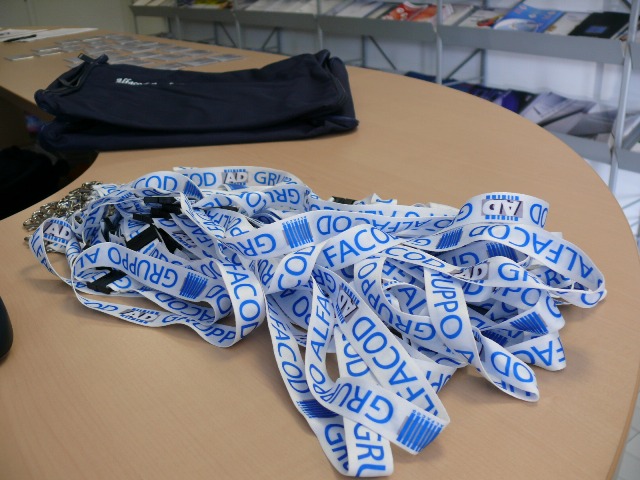The image features a detailed indoor scene centered around a large, oval-shaped tan table that appears to be part of an organizing station. The table surface is occupied by a chaotic pile of white lanyards adorned with light blue text, though the words are mostly obscured due to the tangled arrangement. Among the barely legible text on the lanyards, the initials "G-R-U-P-P-O" and "A-L-F-A" can be discerned. Behind the lanyards, a couple of folded black bags with small white emblems or symbols are positioned. Further back, lining a white wall, are grey shelves connected by poles, filled with items like magazines, books, or pamphlets. Additional objects, possibly name tags or badges, a piece of paper, and a pen, are scattered on the table, suggesting a sign-in area. The table design includes a cut-out section, creating a space where someone can sit or stand while engaging with others across it.